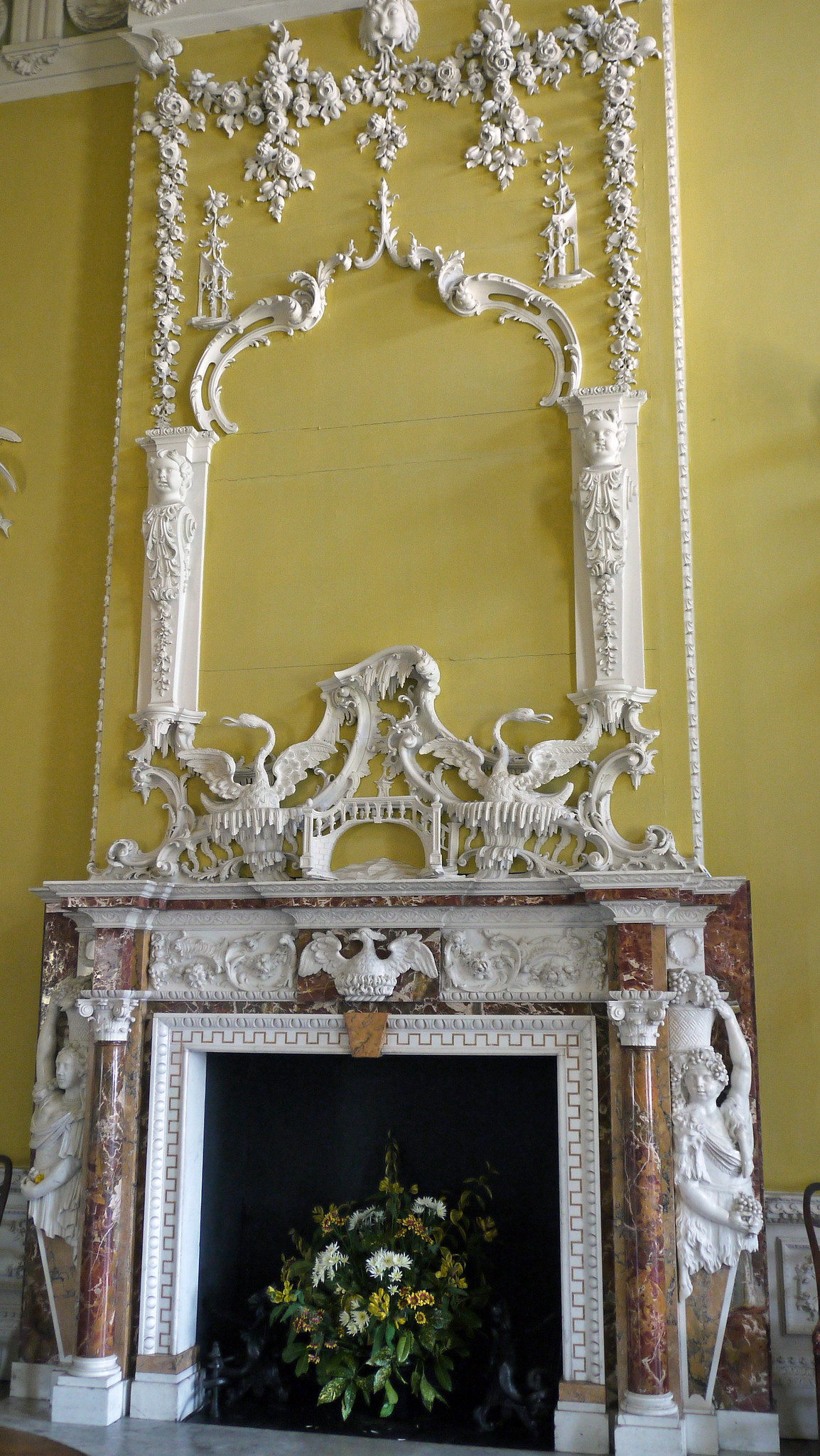The photograph captures an extraordinarily ornate fireplace, likely evoking the grandeur of a castle. The fireplace itself is elaborately decorated with carvings, which include intricate white patterns that look like carved ivory or something similar, set against a backdrop of brown marble, tan, red, and beige hues. The inside of the fireplace, now painted black, is repurposed to hold a stunning bouquet of green and floral arrangements. Flanking the fireplace are partial statues of women, possibly cherubs or angels, seemingly holding up bunches of grapes.

Above the fireplace, an eagle or bird carving draws the eye, serving as an exquisite focal point. The wall behind the fireplace is painted a light olive green-yellow, adorned with matching ornate white decorations that extend all the way up to the ceiling's crown molding. These intricate details include depictions of birds, animals, faces, and an arch adorned with fruit and flowers cascading down, further enhancing the opulent aesthetic. The scene is completed with hints of additional decor, such as pillars, vines, and potentially candles, creating a grand, cohesive design that emphasizes both luxury and attention to detailed craftsmanship. The color palette throughout the scene includes prominent uses of black, white, yellow, brown, and green, enriching the visual complexity and elegance of the room.